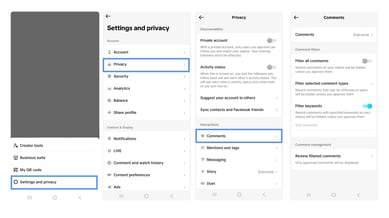This image is a composite screenshot of several screens from a cell phone, organized to create a tutorial-like page for teaching users how to navigate their cell phone's privacy settings. In the upper left-hand corner, there is a blank gray area. Just below and to the right of this gray space, the screen shows a highlighted "Settings and Privacy" menu, specifically with the "Privacy" option selected.

Moving further to the right, the next screen displays the "Privacy" menu, detailing various privacy settings. Part of this screen is blurry, but it is still evident that one of the sliders, possibly related to comments, is turned on and highlighted in teal, while the top slider is turned off.

Below this, a section of the image is outlined with a navy blue box, emphasizing the "Settings and Privacy" menu once again. Following this, there are additional screens; one unmarked, and another highlighting the "Comments" section once again. The final screen in the series is unmarked, completing the visual guide for navigating the privacy settings on a cell phone.